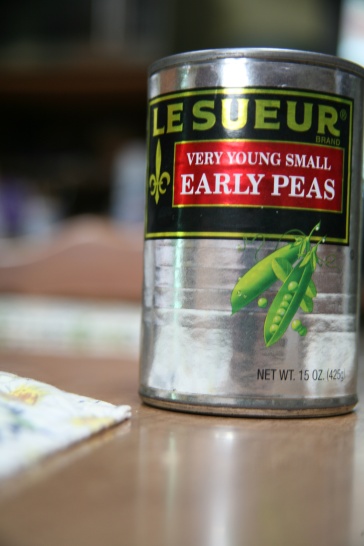A vertical color photo showcases a metal can of vegetables prominently placed on a tabletop. The can, made of standard silver steel, features a detailed label. At the top of the label, set against a black background, the brand name "Le Sueur" is displayed in vibrant green text accompanied by a Fleur de Lis logo. Below the brand name, a white rectangular banner contains the product description in bold white letters: "Very Young Small Early Peas." The label also depicts two green peas, emphasizing the can's contents. Further down, the label indicates the net weight of the can, which is 15 ounces. The background of the image is artistically blurred, keeping the focus entirely on the can of peas.